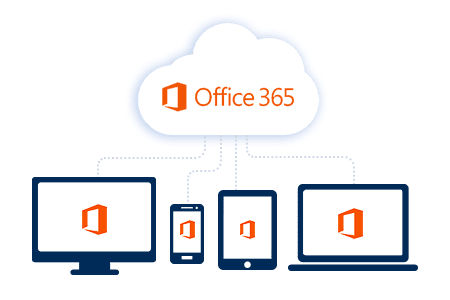This image depicts a family tree-style diagram of Office 365 against a white background. At the center is a stylized, hand-drawn white cloud, not resembling a sky cloud but rather an illustrative one. Inside this cloud is an open, rectangular orange box with the text "Office 365" displayed in a typical Microsoft font. Four lines extend from this central cloud to various devices, representing the "children" of Office 365.

The first device, connected by one of these lines, is an all-in-one computer. It features the orange Office 365 box logo on its screen and appears to have an approximate 18-inch display. The second device is a smartphone with the same logo, resembling a smaller Android phone with a possible 5-inch screen. The third device depicted is a tablet, which could be a Windows, Android, or even a smaller iPad given its mid-size and centrally located button. Finally, the diagram shows a laptop, also featuring the Office 365 logo and resembling an average-sized model.

Overall, the drawing uses size-appropriate illustrations to represent the all-in-one computer, smartphone, tablet, and laptop, each linked back to the central Office 365 cloud.